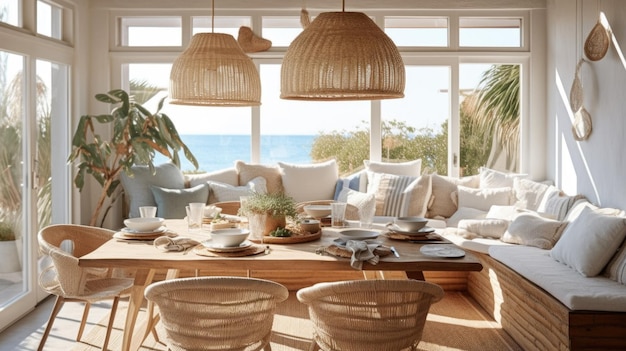The image depicts a beautiful dining room inside a house by the beach, with floor-to-ceiling glass windows providing a stunning view of the aqua-blue ocean and white sky. The room features an abundance of natural light, enhancing the cozy, inviting atmosphere created by the warm, wooden and wicker furnishings. Along the windowed walls, an L-shaped wooden bench with cushions forms a comfortable nook for seating, wrapping around a light brown wooden dining table. Adorning the table are white plates, bowls, silver napkins, and a center platter with a plant, set for a meal. Above, dome-shaped wicker pendant lights hang from the ceiling, casting a soft, beige glow over the setting. On the right wall, there appears to be a bird statue, adding a whimsical touch to the decor. Additionally, there are patio doors on the left side, leading to the beach, with plants visible through the glass, blending the indoor and outdoor elements seamlessly.